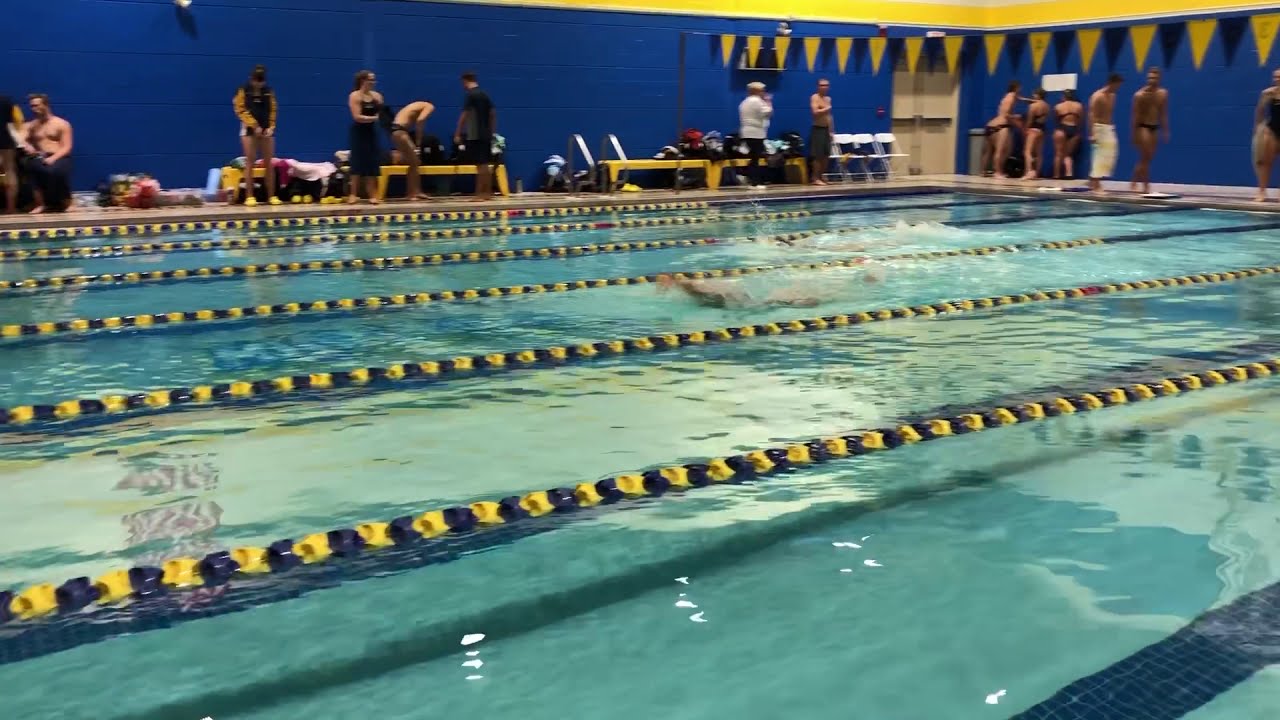The image depicts a bustling indoor swim meet set in a professional-looking swimming pool. The pool itself has six clearly visible lanes, each separated by floating dividers in vibrant yellow and blue. Yellow triangular flags stretch across the pool, adding a festive touch to the scene. The pool floor is adorned with bright blue mosaic tiles, and the water appears crystal clear, reflecting the powerful overhead lighting. The walls in the background are painted in striking red and blue hues, enhancing the vivid atmosphere. On one side of the pool, shirtless men in swim trunks or speedos prepare for their events, with one draped in a towel. On the other side, women can be seen, though it's unclear whether they are in swimwear or casual attire. Despite the poor image quality, a multitude of swimmers—over ten—are discernible, all poised to compete. The photo's focus appears to be on the pool and the swimmers with a particular emphasis on one swimmer prominently visible in the center.